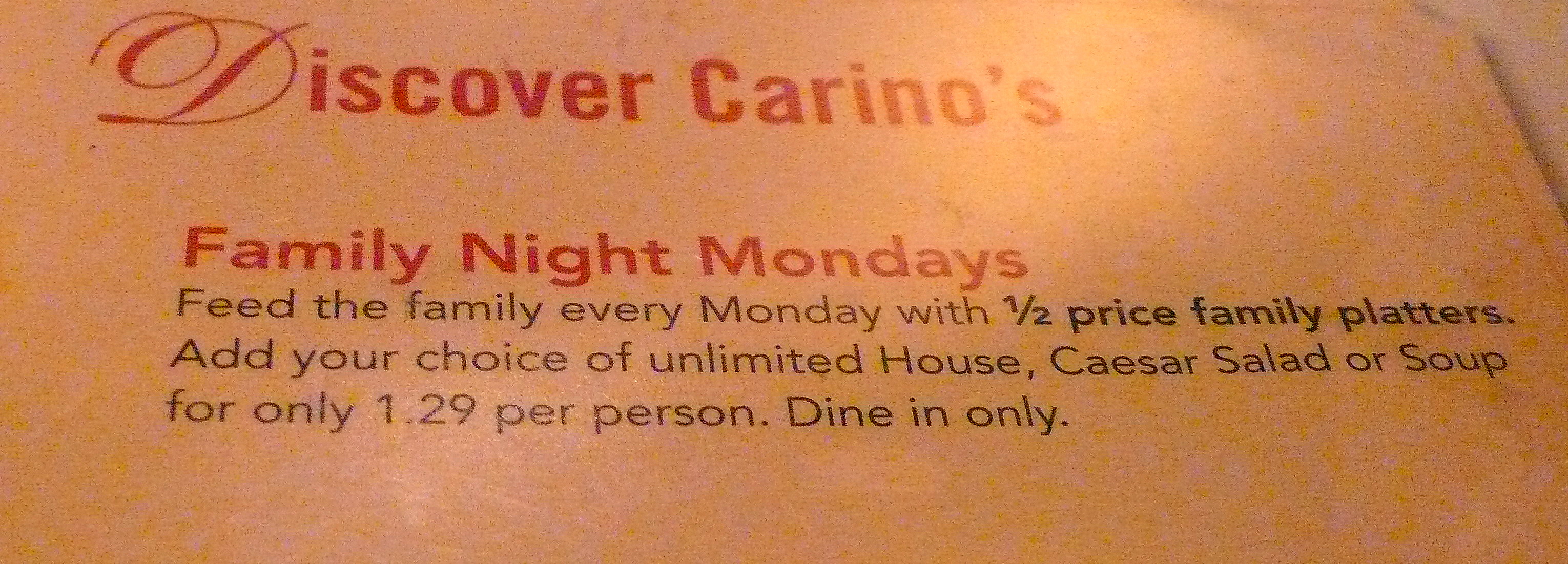The image captures a menu advertisement for Carino's Family Night Mondays, promoting their special dine-in offer. The menu description, printed on a faded orange paper with a slight yellow tinge from the lighting, highlights that every Monday, families can enjoy 'half price family platters' with this offer prominently emboldened in black text below a heading in red. The advertisement also features the detail that patrons can add their choice of unlimited house, Caesar salad, or soup for just $1.29 per person. Despite the slight blur, the text remains legible, and the word "discover" at the beginning of the description is written in a distinctive classical script font, particularly notable in the stylized letter "D." The menu lies atop what seems to be a bare table, adding a cozy, homey ambiance to the scene.